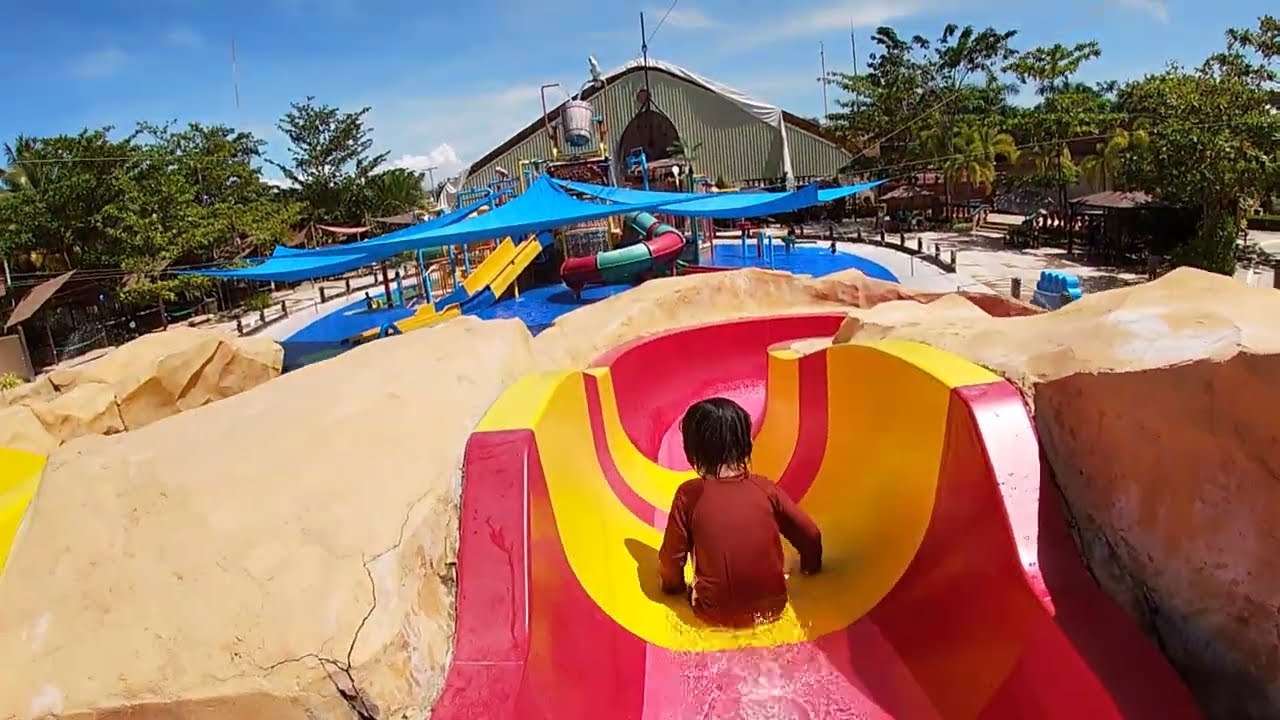In this vibrant outdoor image, a young child with dark hair, dressed in red, sits at the front and center, ready to plunge down a striking yellow and red water slide. The slide, enveloped by rock formations, has splashes of water around it, accentuating the thrill of the ride. The child appears poised on a red and yellow circular buoy, adding a burst of color to the scene. Surrounding the main slide are multiple other vividly colored slides, including teal and pink, and blue and yellow. A blue canopy partially obscures the background slides, adding layers of interest to the image. Behind these features, an odd-shaped, mint-green building stands out against a backdrop of lush green trees and a bright blue sky sprinkled with white clouds. The combination of natural and man-made elements, along with the array of bright colors, makes this water park scene lively and dynamic.